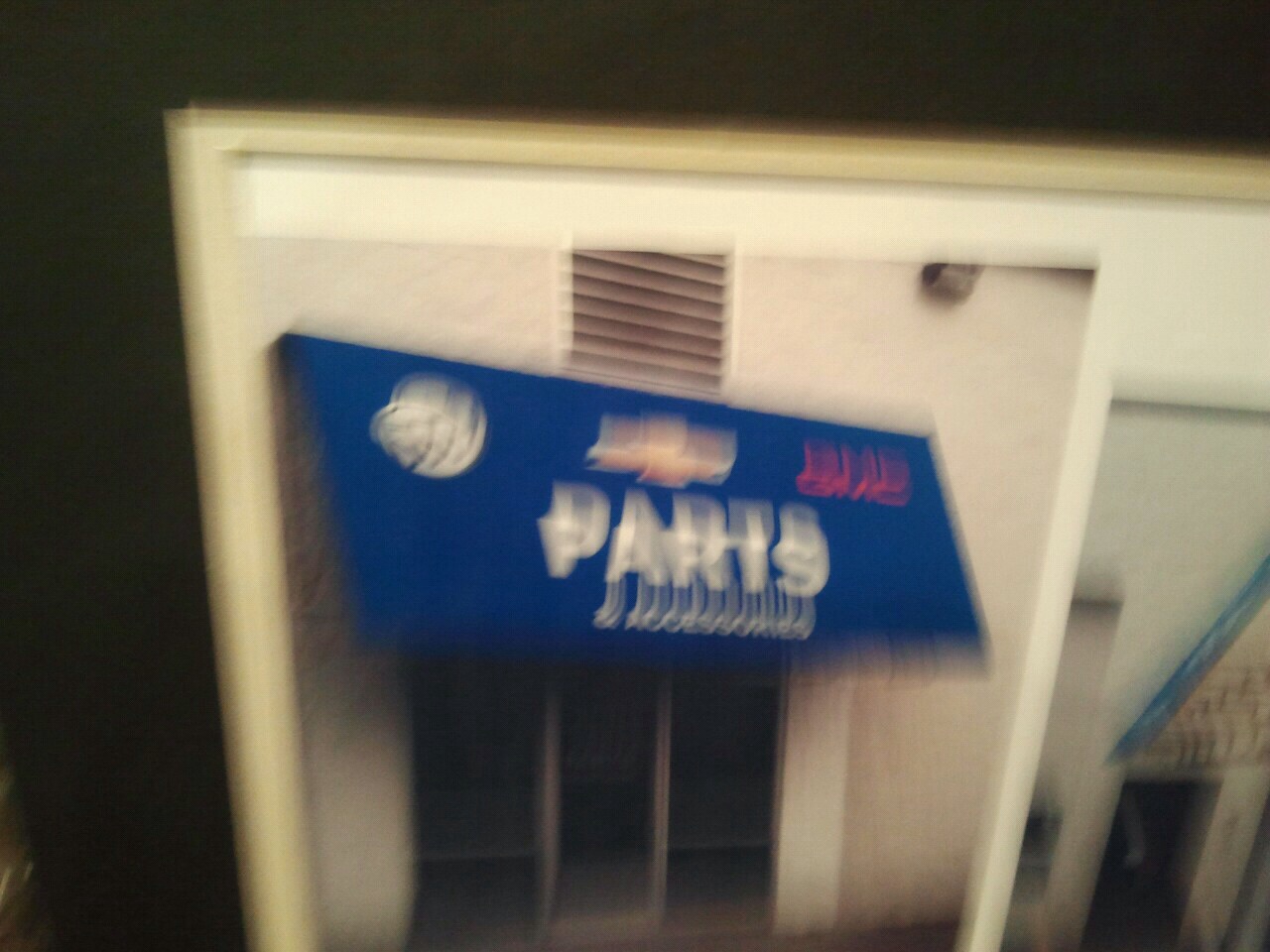The photograph captures a pair of shopfront images encased within a border. Unfortunately, the central photograph is very blurry, with a vertical blur evident throughout the image. On the left side of this blurry photograph, a shop is discernible, characterized by the word "parts" displayed prominently in white text. Further details include a white object in the top left corner, a Chevrolet emblem centered at the top, and a red GMC logo situated at the top right. The shop itself features a blue canopy, complemented by visible glass windows and a vent positioned at the very top. Conversely, the right side of the image depicts a white wall crowned with a blue rooftop. The overall visual comprises shopfront scenes, denoting commercial storefronts.